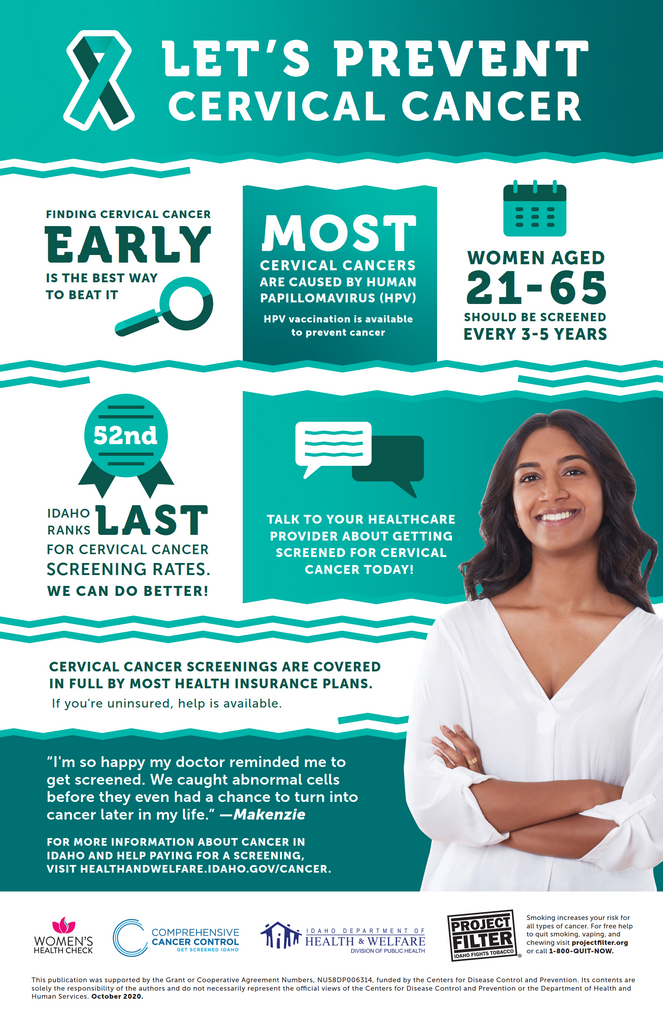The poster, designed in a green and white color theme with occasional blue and pink accents, provides detailed information about preventing cervical cancer. Positioned prominently at the top, the message "Let's prevent cervical cancer" is written in bold white letters against a green background. Below this, essential points highlight the importance of early detection and regular screenings, stating that finding cervical cancer early is crucial, with a magnifying glass icon emphasizing the point. It mentions that most cervical cancers are caused by HPV and that HPV vaccination is available to prevent it. A blue-bordered calendar icon notes that women aged 21 to 65 should be screened every three to five years.

In the bottom right corner of the poster, there's an image of an African-American woman with long black hair wearing a white top with a plunging neckline, her arms crossed at her waist. Below her image, a green rectangle contains a quote about how her doctor helped her by catching abnormal cells early. The poster also underscores that Idaho ranks low in cervical cancer screening rates, encouraging women to talk to their healthcare providers. It affirms that cervical cancer screenings are covered by most health insurance plans and that help is available for the uninsured.

At the bottom of the poster, logos and names of organizations, including Women's Health Check, Comprehensive Cancer Control, and the Idaho Department of Health and Welfare, are displayed, mainly in blue and pink. The poster concludes with a call to action: "Get screened, Idaho." For further information, individuals are directed to visit health and welfare websites. This comprehensive poster aims to raise awareness and encourage proactive health measures to combat cervical cancer.